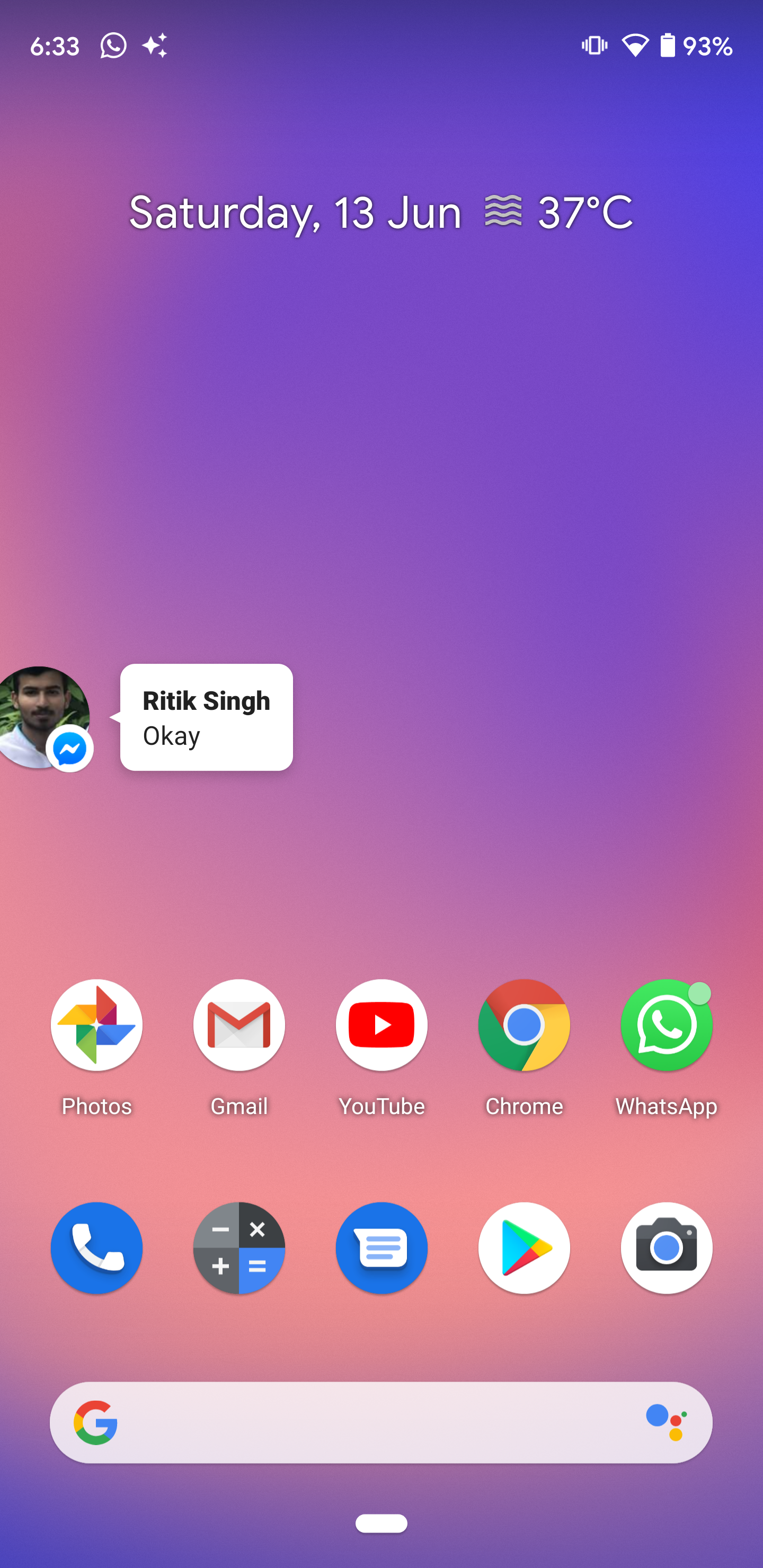The image showcases the user interface of Smiley's phone. In the top left corner, the time is displayed as 6:33. Adjacent to the time, on the right, there are a few icons, and further to the far right, the Wi-Fi icon and a battery indicator showing 93% battery life can be seen. 

The background features a gradient that starts with a blue hue at the top right and gradually shifts through shades of magenta, pink, and purple as it descends. Centrally situated near the top, the text displays the date and weather: "Saturday, 13 June - 37°C". Below this text is a small profile picture of a man with a mustache, wearing a light-colored shirt, positioned to the left. The name "Rateek Singh" accompanies the profile picture, alongside a text box containing his comment: "ok".

Below Rateek Singh's comment, there are ten different icons arranged presumably for various phone functions. At the very bottom, a Google search bar is prominently placed for quick access.